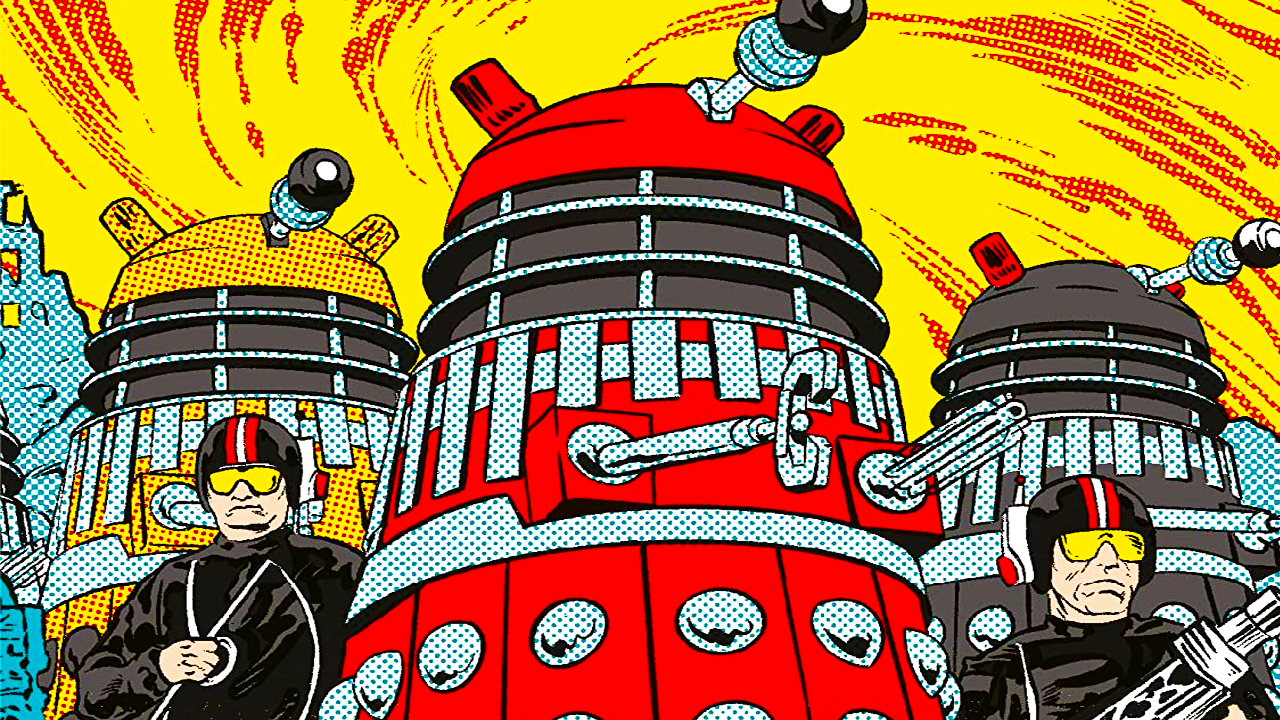In this vintage 1950s-style cartoon illustration, the focal point is a trio of tall, oblong robots. The central robot, red and resembling a trash can, features silver metal studs, a claw-like arm, and a blender-like appendage. Similar robots flank it: a yellow one on the left and a dark gray one on the right. Each robot has a speaker-like element on top. The sky is a swirling mix of yellow and red streaks, adding a dynamic background to the scene. Flanking the robots are two men dressed in black outfits with black helmets adorned with a red and white stripe, and yellow sunglasses. They are each holding weapons, adding an element of tension and action to the image.